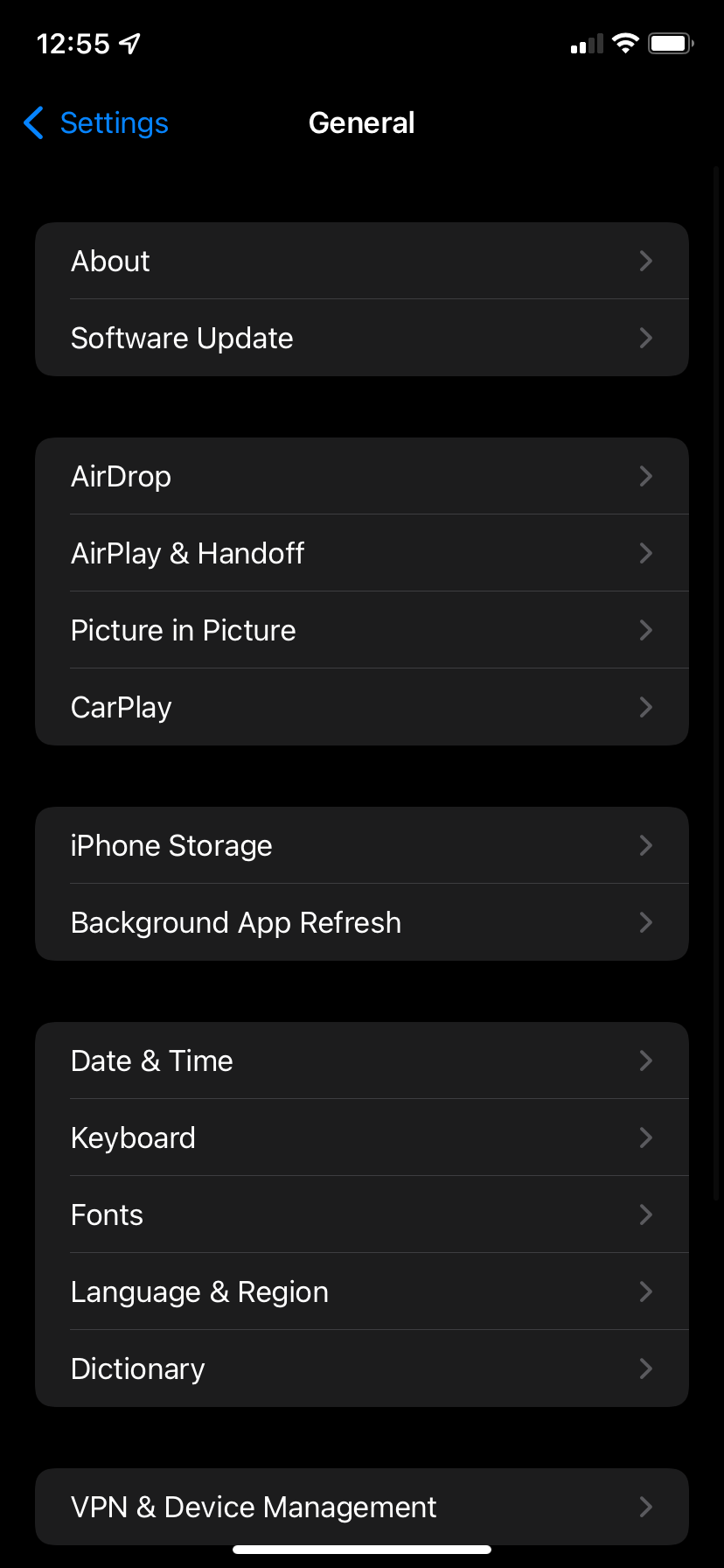A detailed screenshot from an iPhone in the General section of the Settings menu. In the upper left corner, the time is displayed as 12:55, and there is a small arrow icon. The upper right corner showcases icons for signal strength, Wi-Fi connectivity, and battery life. In the center of the top portion, the word "General" is prominently displayed, with a blue "Settings" button to its left.

Beneath the header, various options are listed, each accompanied by a right-pointing arrow indicating the presence of additional sub-menus. The options listed are:

- About
- Software Update
- AirDrop
- AirPlay & Handoff
- Picture in Picture
- CarPlay
- iPhone Storage
- Background App Refresh
- Date & Time
- Keyboard
- Fonts
- Language & Region
- Dictionary
- VPN & Device Management

Each option is enclosed in its own separate box. The text is white, set against a black background, signifying that the device is in dark mode. No other features, functions, objects, or images are present in this screenshot.